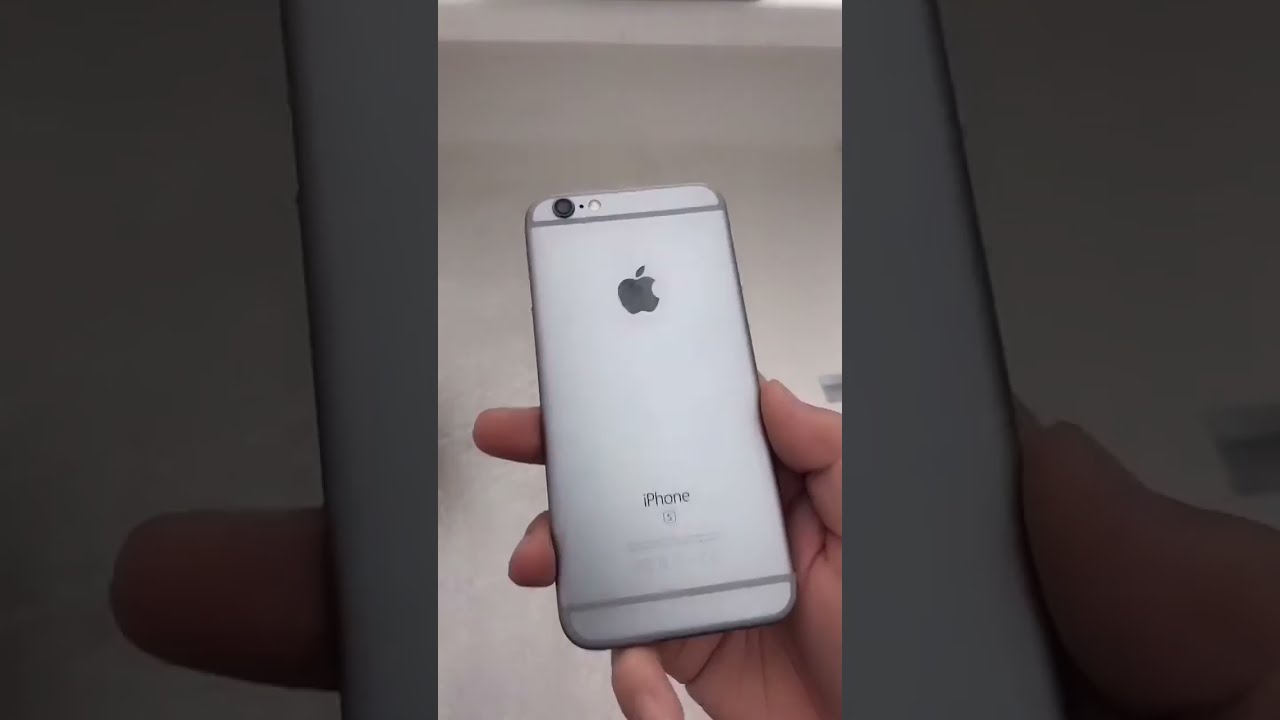The image is a photorealistic composition featuring a close-up of a person's right hand holding a silver iPhone. The central third of the image, extending from the bottom to the top, is in sharp focus, while the left and right thirds show zoomed-in and darkened versions of the same photograph. The iPhone is positioned with its back facing the camera, showcasing a black Apple logo near the top center and the word "iPhone" with a small "S" near the bottom. The phone features a black camera lens with a flash at the top left corner. The background appears to be a light gray or beige wall, possibly tile or concrete, with a white line running across the top. The hand holding the phone is a Caucasian male's right hand, with the thumb and index finger gripping the sides and the other fingers slightly bent. The overall effect creates a layered visual experience, with the central, vibrant image standing out against the darker, blurred background versions.